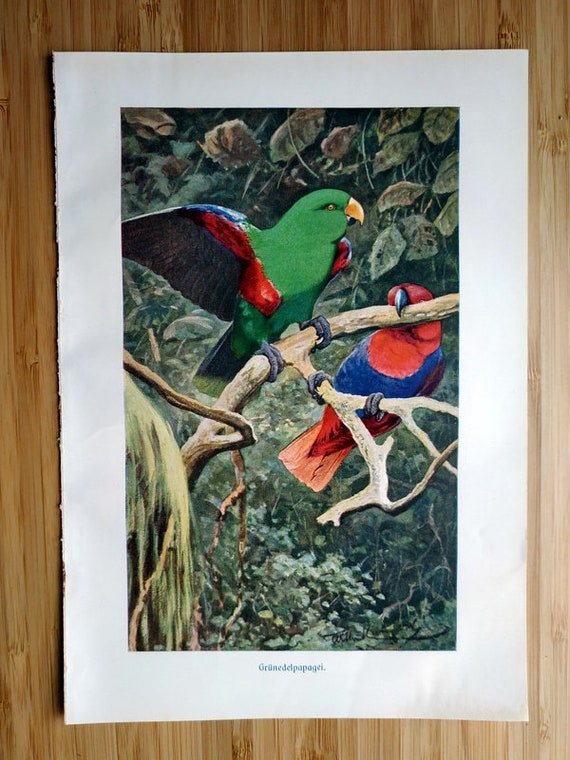The image features a framed piece of artwork on a light tan wooden wall. The frame is made of brown wood and the artwork itself is bordered by a white margin. The artwork depicts two colorful birds, which resemble parrots or cockatoos, resting on a wooden branch that stretches from right to left and branches off in the middle. The scene is set against a backdrop of green leaves and bushes, with some brown leaves also visible.

One bird, vibrant in green, has an orange beak, red and blue wings with blue tips, black underwings, black feet, and a gradient tail that transitions from light green to dark blue. This bird is perched securely on the branch. The second bird, which is red and blue, has a red head, neck, and chest, with the red extending partly into the midsection, which then transitions to a dark blue body. Its feet are blue and its beak is black. It perches on the branching-off part of the branch, holding onto it with both its beak and talons. Below the artwork, there's a piece of print text that is too small to read.